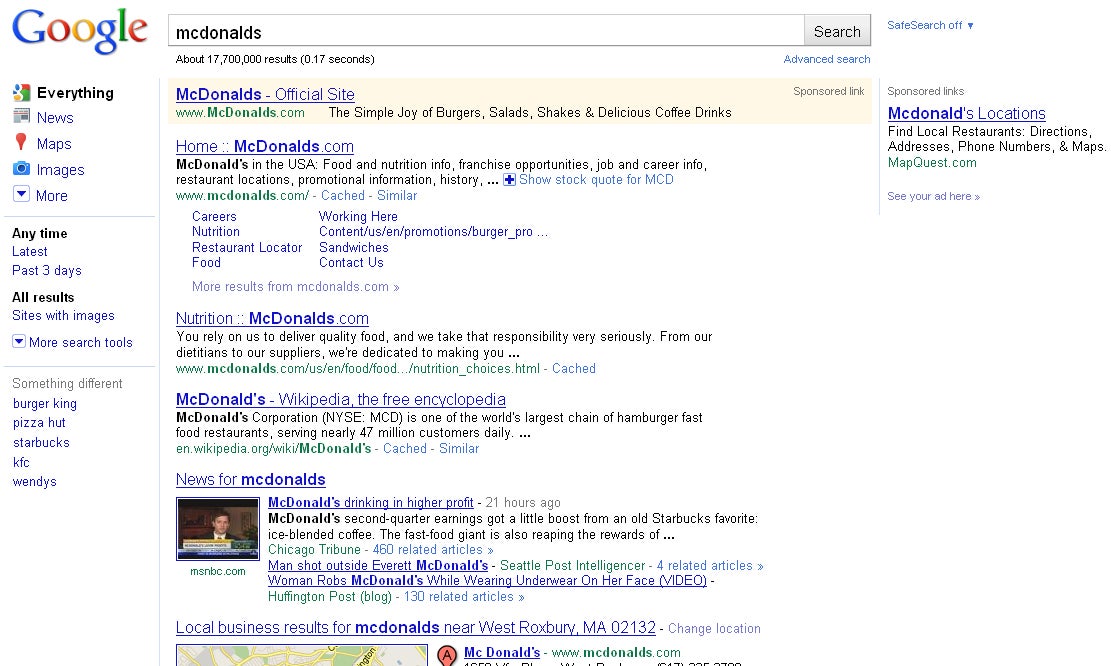The image features a Google search results page for "McDonald's." 

At the top left corner, the familiar Google logo is displayed next to a prominent search bar. Within the search bar, the term "McDonald's" has been entered. Directly adjacent to the search bar on the right is a search button. 

On the left side of the page, a vertical toolbar provides multiple filter options such as "All," "News," "Maps," "Images," and "More." Below these options, additional filters like "Anytime," "Latest," "Past 3 days," and "All results" can be found. The toolbar also includes advanced search options like "Sites with images," "Airplane," and "More research tools." 

The main section of the page shows the search results. At the top, a sponsored link for McDonald's official website is displayed, featuring the URL "mcdonalds.com" and various sections such as "Home," "Nutrition," and "Promotions." The description under the link provides detailed information about McDonald's in the USA, covering elements like food nutrition, franchise opportunities, job and career information, restaurant locations, promotional information, and history. 

Below this sponsored entry are additional blue hyperlinks leading to various sections of the McDonald's website, including "Careers," "Working Here," "Nutrition Content," "Promotion," "Burger Restaurant Locator," "Sandwiches," "Food," and "Contact Us." 

On the right side of the search results, there is another sponsored section highlighting "McDonald's Locations," which provides further information under each link. Finally, the "News" section showcases a small image associated with a recent news story about McDonald's.